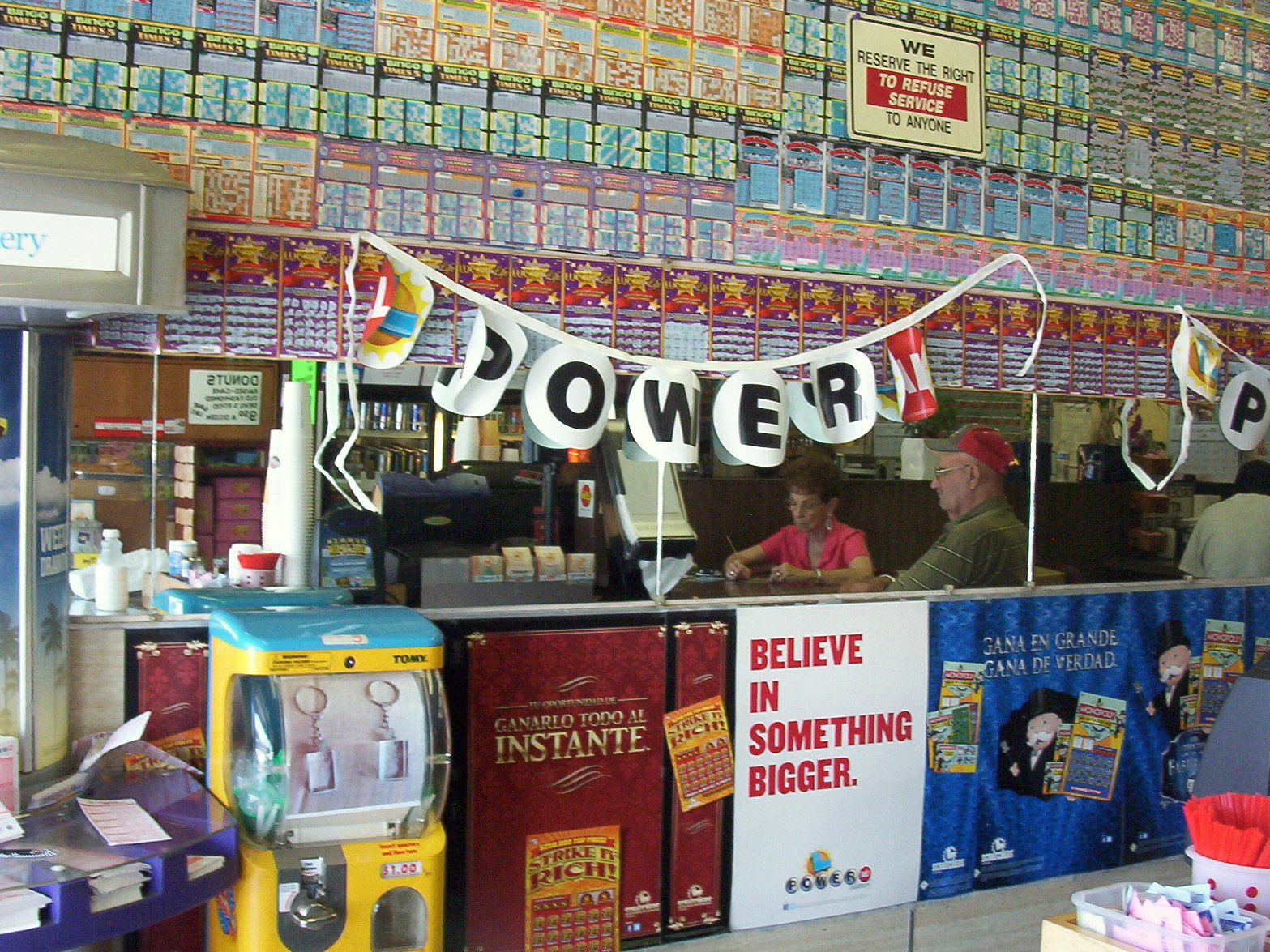The image depicts the bustling interior of a small lottery shop, with a counter at the center of the scene. The shop is adorned with numerous eye-catching details. Along the top of the wall, rows of colorful lottery scratch-off tickets are prominently displayed, some of them featuring Spanish phrases like "ganarlo todo al instante," "Ghana en grande," and "Ghana de verdad." Above these tickets, a white sign with black text declares, "We reserve the right to refuse service to anyone."

A white strip of paper bearing the word "POWER," with each letter encircled and pasted on it, acts as a cheerful streamer hung alongside a larger Powerball banner. The front of the counter is festooned with multiple banners promoting different scratch-off tickets.

At the counter, a woman clerk, dressed in a pink top, is engrossed in writing something with a pen. In front of her is a box of tissues and a variety of notices. Nearby, a man in a green shirt and a red-and-green ball cap stands waiting, suggesting a transaction in progress. In the bottom left corner, a yellow and blue gacha machine is visible, adding to the store’s eclectic charm. The vibrant setting, filled with advertisements and promotional banners, vividly captures the lively atmosphere of the lottery shop.